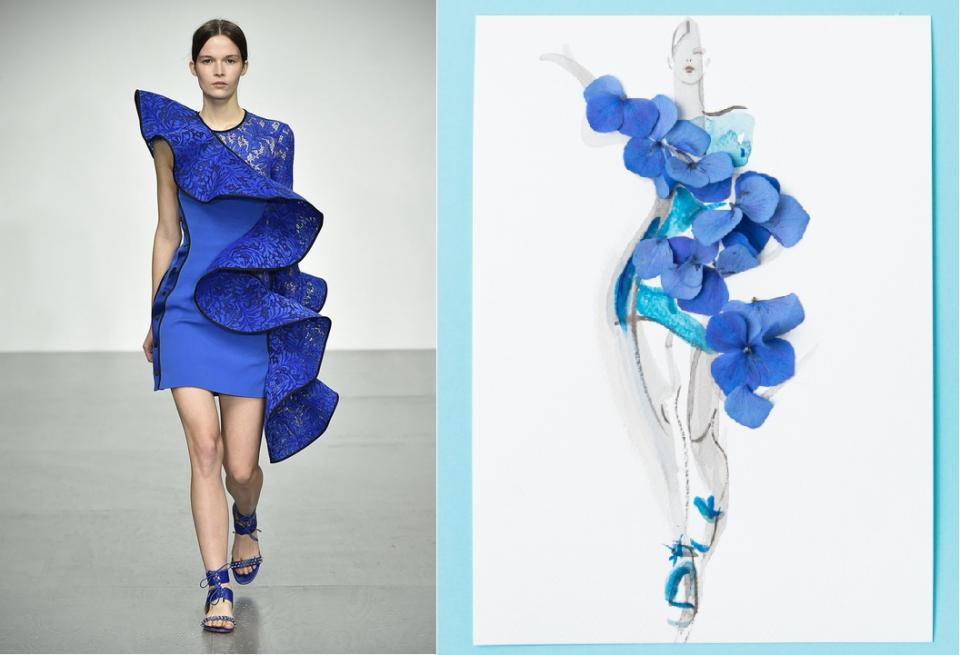The image consists of two parts side-by-side. On the left is a photograph of a model strutting down a light gray runway with a white backdrop. She has black hair parted in the middle and tied into a ponytail, and she's wearing a striking blue dress. The dress features a large, wavy, protruding fabric that starts at her right shoulder and elegantly cascades down to her left side, giving it an oversized, artsy look. The garment is complemented by strappy blue heels. On the right side, there is a sketch that conceptually explains the design of the dress. The sketch is a simple illustration of a woman in a blue dress, but with an additional layer of mixed media showing blue flower petals, which represent the wavy fabric seen on the actual dress. The sketch provides clarity and enhances the overall design, suggesting an idealized version of the dress seen on the left.